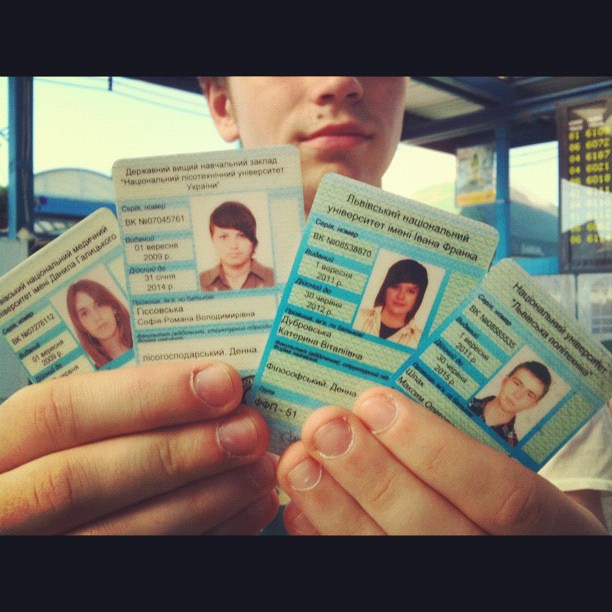In this photo, a young man with a fair complexion is seen holding up four IDs, partially obscuring his face from the nose upward. Notable on his visible face is a small mole above his left upper lip. The IDs he is holding are adorned with photos and text in the Cyrillic alphabet, suggesting Russian or a similar language. The IDs feature the pictures of multiple people: at least one male and several females. The scene is set in an indoor environment, possibly a structure with windows that provide a view of the outside, though the specifics cannot be discerned. The surrounding background includes blue bars and a poster with yellow lettering. The image is bordered by a black strip at the top and bottom.